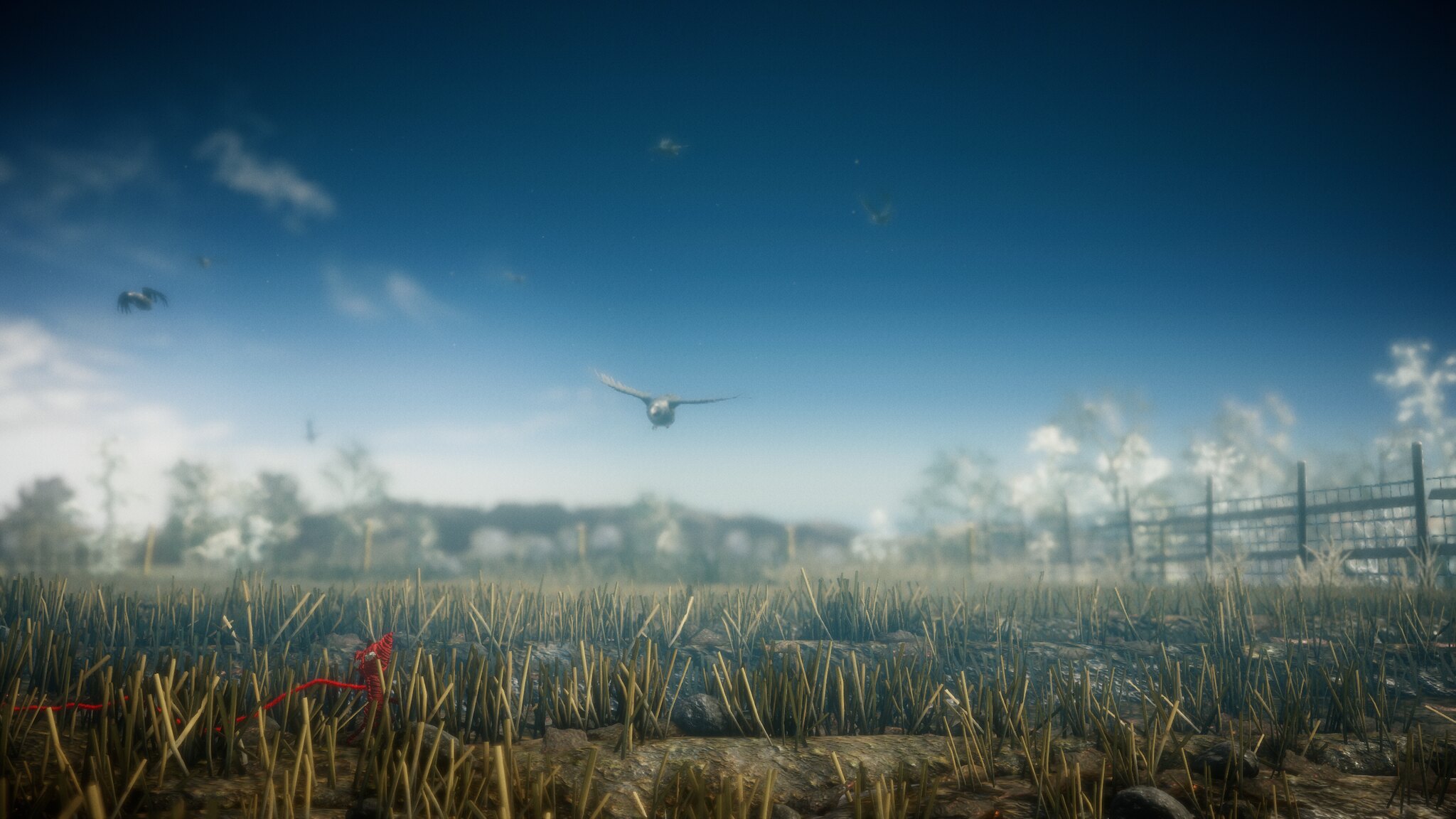This computer-generated-looking image captures a serene outdoor scene of a vast field with sparse dirt and patches of grass. A distinctive, complex fence structure is visible on the right side; it consists of a black, horizontal-plank fence that overlays a larger mesh of small squares. The ground is primarily brown with small yellow and tan protrusions, possibly new grass, and scattered with pieces of a long red ribbon. In the sky, which transitions from dark to light blue as it approaches the horizon, there are fluffy white clouds and two birds in flight. The bird closer to the camera has a wide wingspan and gray and white feathers, resembling a hawk, while the more distant bird appears black and white in silhouette. A row of trees or possibly a grove is barely visible in the blurred distance, adding depth to this tranquil scene.